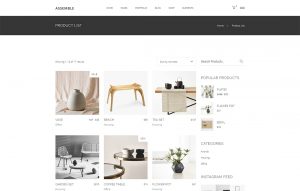The cropped screenshot of an online store showcases a visually appealing yet slightly disorganized layout. The primary navigation tabs are positioned at the top of the page, featuring black text on a white background. Just below this, there is a secondary navigation bar with three tabs against a black background – one on the top left and two on the top right, labeled "Log In" or "Sign In."

The main content area of the webpage, which also has a white background, displays various products. On the left side, there is a cream-white pot plant. Directly below it, a set of grey chairs is positioned around a white and grey table. The room's background is a subtle grey, with a pristine white floor enhancing the clean and modern aesthetic.

To the right of the pot plant sits a wooden table in a rich brown hue. Adjacent to this table, there is another table draped with a light brown fabric, further adorned with brown-toned pot plants. In the bottom right corner of the image, a black pot plant containing a vibrant green plant catches the eye. To the left of this black pot, a table with a glass top and a slightly cream-white backdrop adds diversity to the furniture display.

Numerous additional products are visible on the right side of the image, including various pot plants. However, due to the image's small size, the accompanying text is blurry and unreadable, leaving some details unclear.